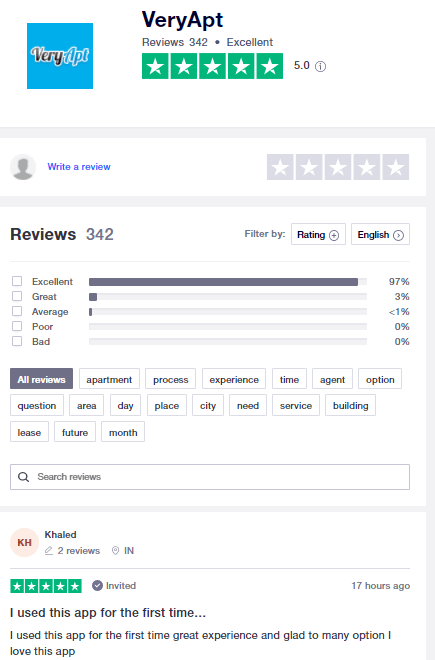The image captured on a mobile phone depicts an apartment review website named Very Apt. The platform, possibly also known as Very Apartment, currently hosts 342 reviews and boasts an impressive 5-star rating. Review categories available to users include: Excellent, Great, Average, Poor, and Bad. Notably, the majority of reviewers selected 'Excellent,' with very few choosing 'Great' or 'Average,' and none opting for 'Poor' or 'Bad.'

Users can filter reviews by several distinct categories, such as: All Reviews, Apartment Process, Experience, Time, Agent, Option, Question, Area, Day, Place, City, Need, Service, Building, Lease, Future, and Month. Additionally, there's a 'Search Reviews' function below these categories.

The showcased review is authored by a user named Khaled from Indiana, who has contributed two reviews in total. Invited to use the app, Khaled shared their feedback just 17 hours ago, awarding a 5-star rating and commenting, "I used this app for the first time. Great experience, glad to see many options. I love this app."

The entire review interface is set against a plain white background and is displayed in a vertical portrait orientation.